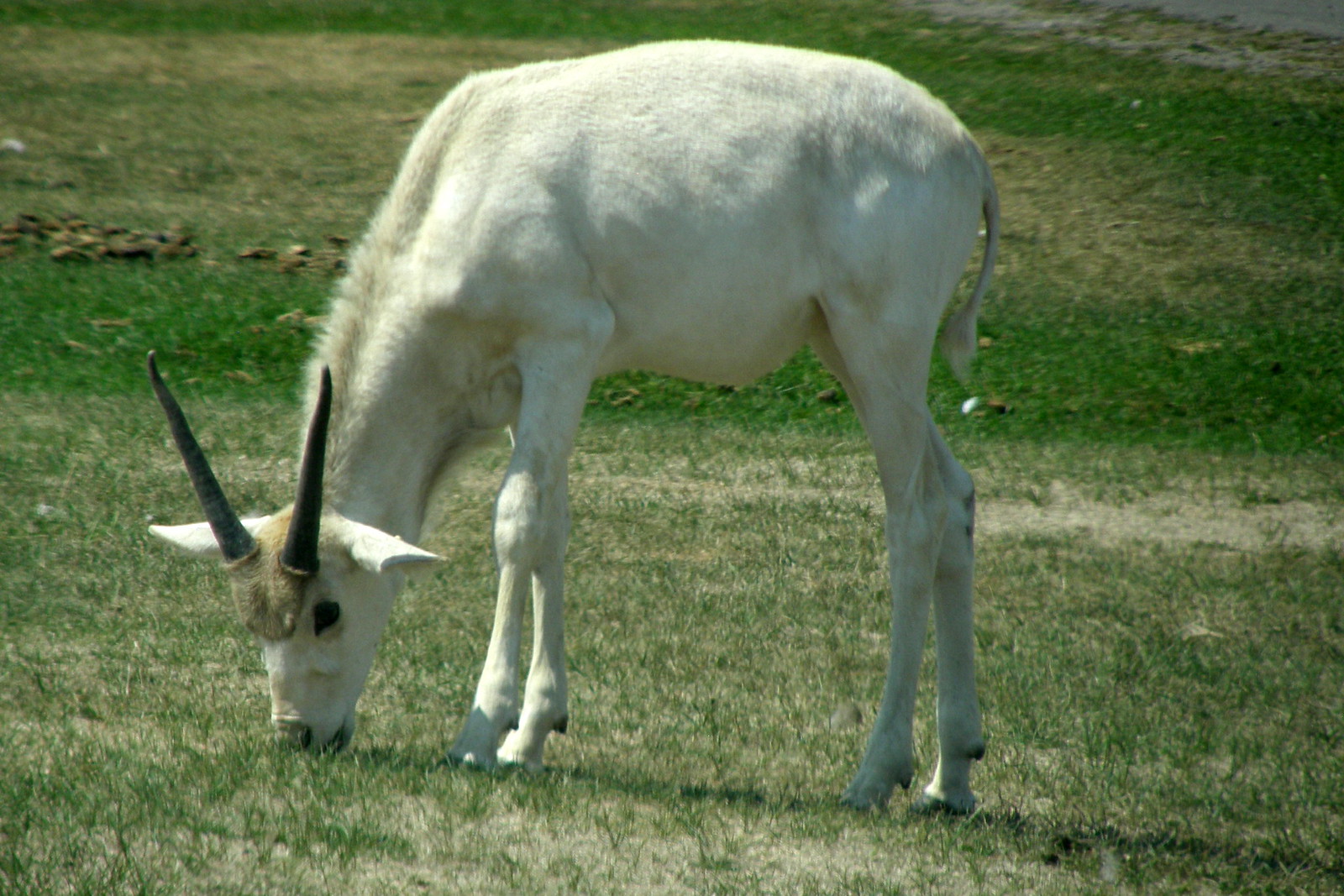The photograph captures a baby addax, a species also known as the white antelope, native to the Sahara Desert. The young addax is centered in the image, grazing on grass in what appears to be an open area, possibly a zoo. With its head lowered towards the ground, the addax's side profile reveals one visible eye and short, straight horns that have just begun to spiral. The baby addax has mostly white fur with patches of brown, especially around its neck and near the horns. It has a long neck, slender legs, and a small tail. The background features a field of predominantly green grass interspersed with some brown patches, dirt, and possibly an asphalt trail in the top right corner, mostly cropped out of view.